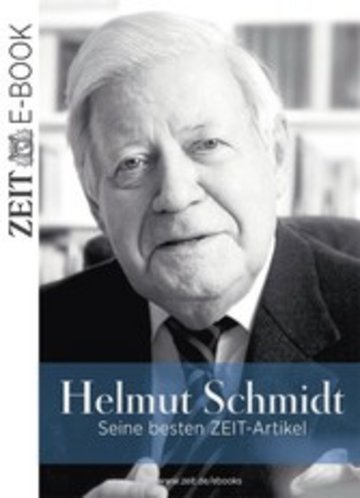The image is a well-centered, black-and-white cover of an e-book featuring an elderly man, approximately in his 70s, with short, combed, white hair. He is staring directly at the camera with a neutral expression, his mouth slightly open. He is dressed in a black suit coat over a white collared dress shirt paired with a black and gray striped tie. His raised hands are visible at the bottom of the cover.

On the lower section of the cover, the text "Helmut Schmidt" is prominently displayed in white letters against a rectangular dark blue background. Beneath his name, another line reads "Sein Besten Zeitartikel" in white, suggesting the language is German. Vertically aligned on the left side, the word "ZEIT" appears in large, all-caps letters, followed by an icon and the word "e-book." The background subtly suggests an office setting, with what appears to be bookshelves behind him, reinforcing the professional and scholarly atmosphere.